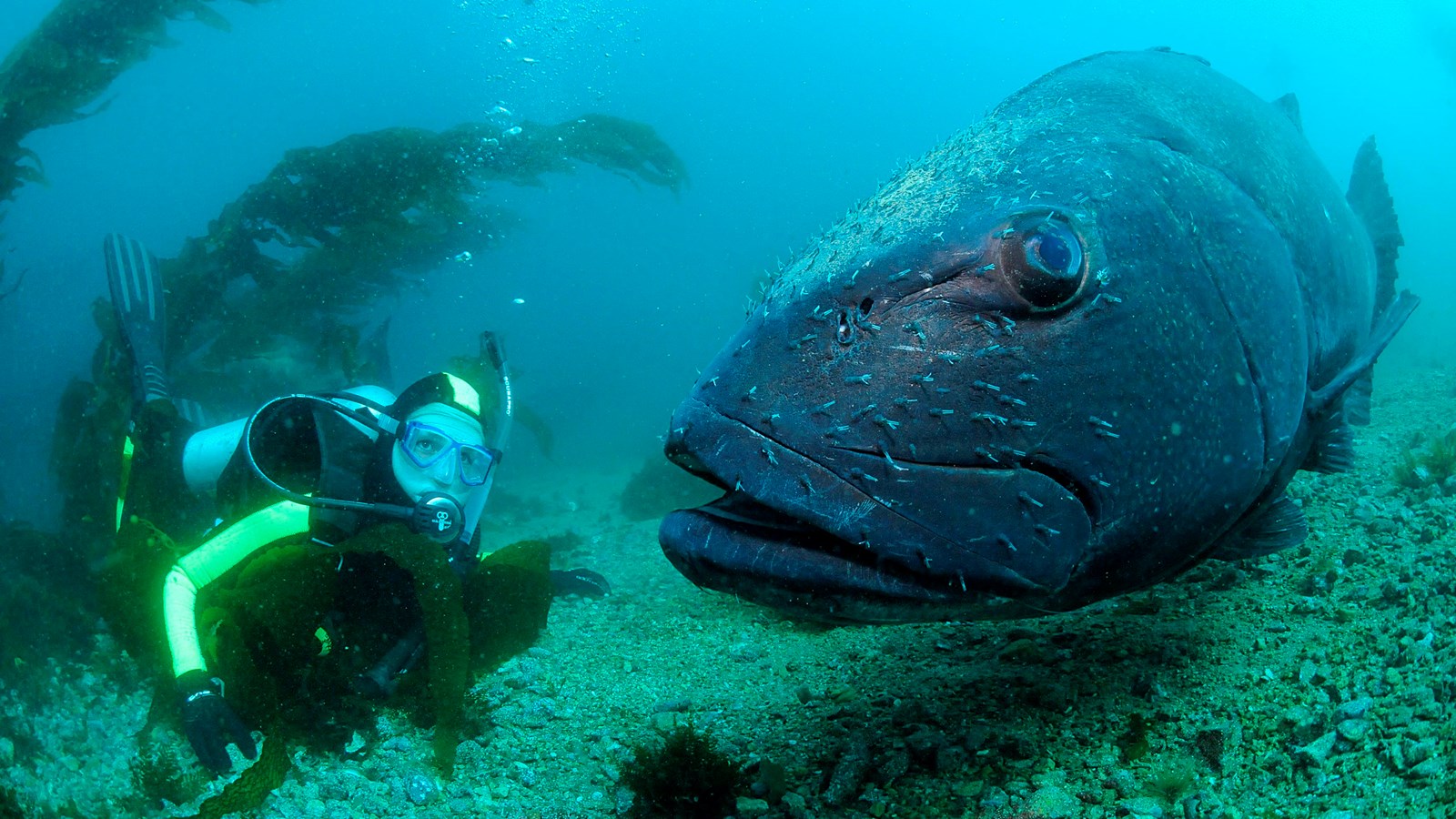This underwater photograph captures a deep-sea diver and a massive, prehistoric-looking fish side by side in a vivid deep-sea environment. The scuba diver, positioned on the left, is wearing a scuba suit accented with bright neon green and black, and is equipped with a light blue oxygen tank. Reflective neon green coatings on his right arm and flippers stand out in the cyan bluish tint caused by the underwater setting. Bubbles emerge from his breathing apparatus, and he appears to be looking directly at the camera. To the right of the diver, the fish, with its large, slightly open mouth and impressive, near-black blue-gray body, gazes toward the viewer with one enormous eye. The background features seaweed behind the diver, while the bed beneath them is strewn with gravelly rocks. The entire scene is bathed in the blue hues of the ocean, enhancing the surreal, almost otherworldly atmosphere of this underwater encounter.